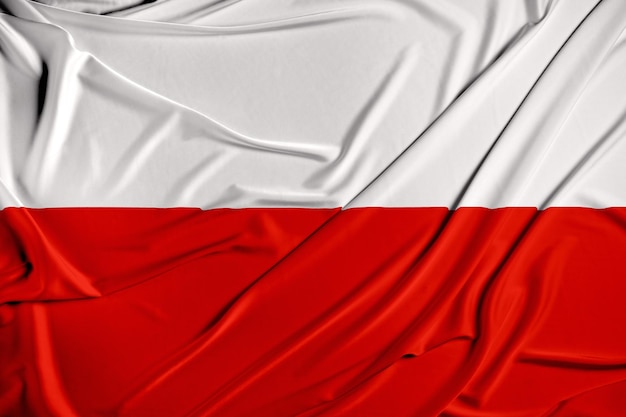This image showcases a striking textile, likely a high thread count sheet or even silk, distinguished by its bold two-tone coloration and detailed texture. The photograph captures the intricate folds and ruffles of the material, emphasizing its luxurious quality. The top half of the sheet is pure white, contrasting dramatically with the bottom half, which is a deep, bold red. The division between these two colors is remarkably straight, though it follows the natural folds of the fabric, creating an intriguing visual effect. The red section appears almost as if a bar has been placed over the material in the image. The sheet, slightly bunched up and wrinkled, runs diagonally from the bottom left to the top right, crossing the image in a long rectangular form. The meticulous depiction of the fabric's texture and the vibrant, clean colors make the sheet appear almost as if it's two separate photographs seamlessly merged.